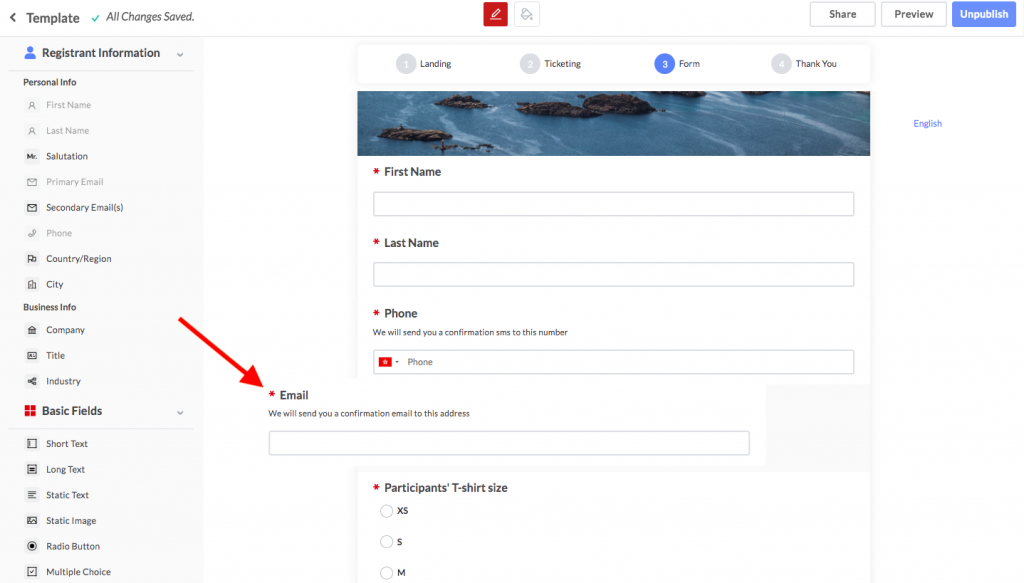The top section of the page features a white and black background with text that reads "Template." There is a green checkmark accompanying the message "All changes saved." Below this header, two boxes are displayed: one red box with a white pencil icon and another box with a white border and an icon depicting a paint can tipping over paint.

At the top right, three boxes are located. Two have a gray outline. The first is labeled "Share" in black text, and the second reads "Preview" in black. The third box, colored periwinkle, features the white text "Unpublished."

On the left side of the page, a gray panel lists several sections in black text: "Registering Information,” “Personal Info,” “First Name,” “Last Name,” “Salutation,” “Primary Email,” “Secondary Email,” “Phone,” “Country/Region,” “City,” “Business Info,” “Company,” “Title,” “Industry,” and “Basic Fields.” Below this, a gray horizontal line separates the panel from a subsequent list: "Short Text," "Long Text," "Static Text," "Static Image," "Video Button," and "Multiple Choice."

Moving to the central section, four clickable segments are displayed with numbers beside them. The first two are gray circles with numbers "1" and "2," labeled "Landing" and "Taking" respectively in black text. The third segment is a blue circle with a white "3" inside it and the label "Form" in black text. The final segment is a gray circle with a white "4," labeled "Thank You" in black text.

An image of an ocean with brown rocks forms a central feature. Below this, fields to capture user information are marked with asterisks: "First Name," "Last Name," and "Phone” with the note "We will send you a confirmation SMS to this number." 

A red arrow points to the field labeled "Email," accompanied by the text, "We will send you a confirmation email to this address." Below, a section marked "Participant's T-shirt Size" has a red asterisk, followed by options for sizes: "Extra Small," "Small," and "Medium."